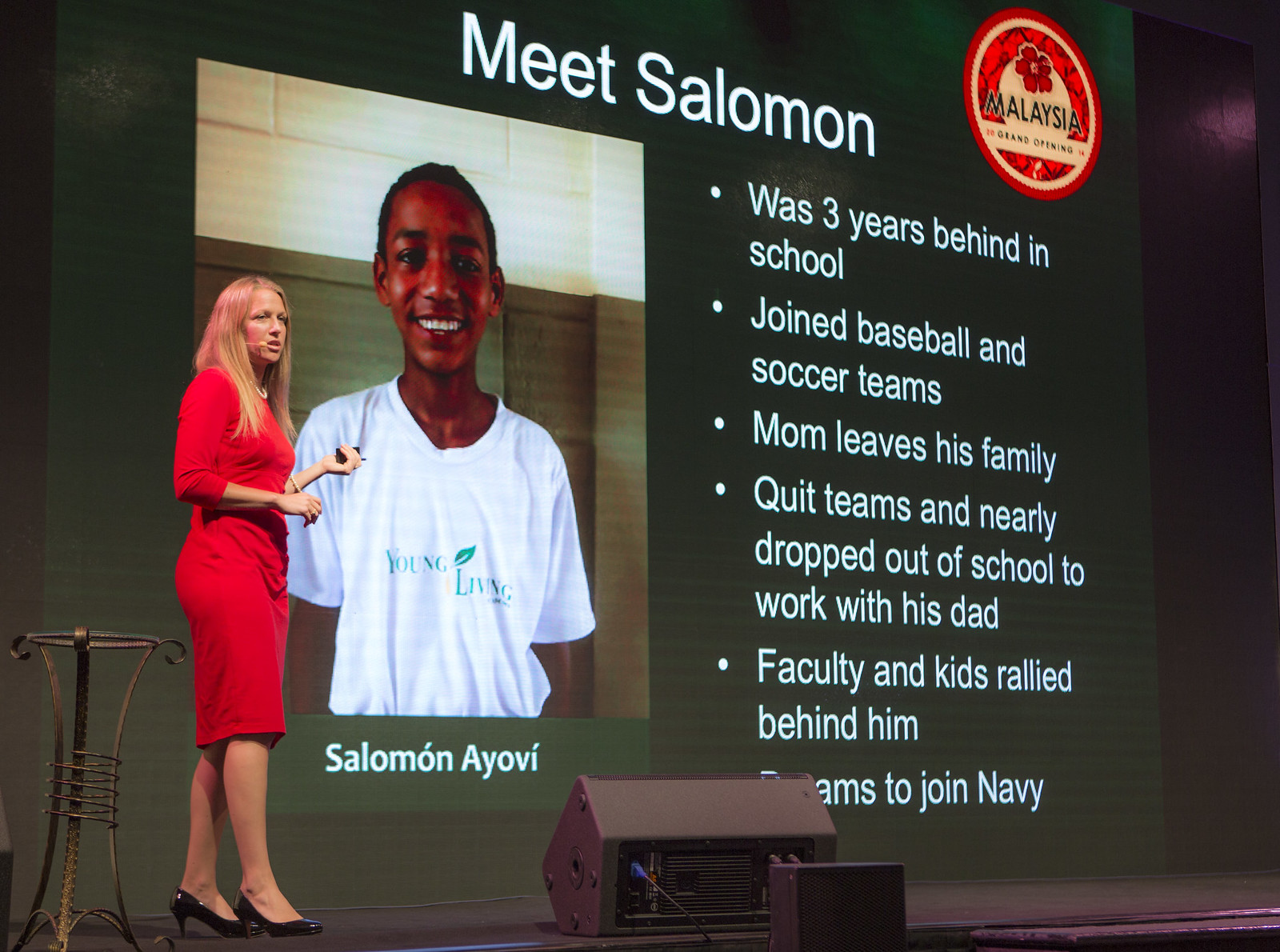In this color photograph, a blonde woman with long, straight hair stands on a dimly lit stage, facing an unseen audience. She is dressed in a striking red dress paired with black high heels and is wearing a small, beige head mic hooked over her ear. Behind her, a large screen dominates the background, displaying the headline "Meet Solomon" in white letters against a dark backdrop. The screen features a prominently placed photograph of a smiling young boy in a white t-shirt with a logo on it. Alongside his image, additional details are presented in bullet points: he was three years behind in school, joined baseball and soccer teams, faced family challenges when his mother left, quit the teams, and nearly dropped out to work with his father. The faculty and students rallied to support him, and there is a note about him joining the Navy, although it's partially obscured. The stage atmosphere is very dark, enhancing the contrast of the white text and the image behind the speaker.